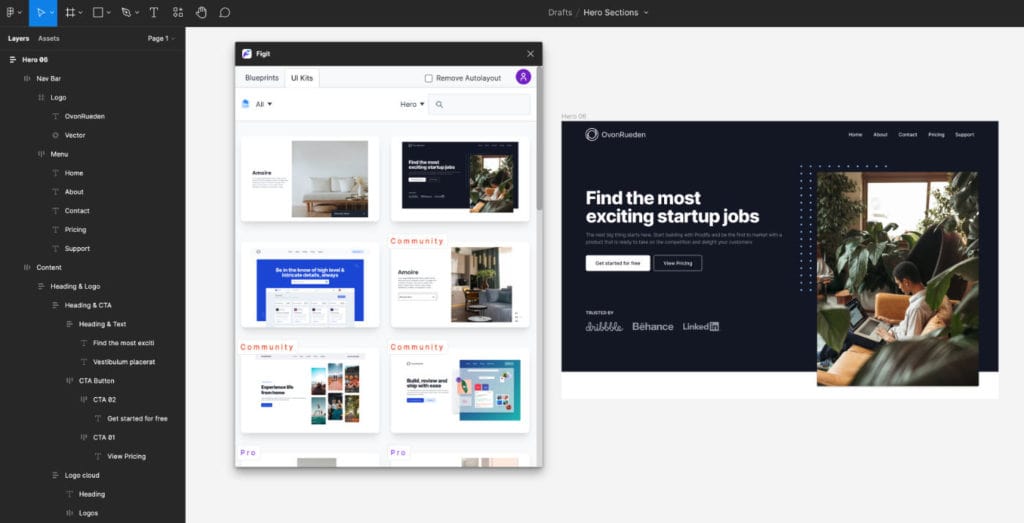In the center of the image, prominently on the right side, there is a black text that reads "Oven Roden" against a dark blue background. Below this text, a tagline encourages viewers to "find the most exciting startup jobs." This tagline is followed by two buttons: one labeled "Get Started" in white and another labeled "View Pricing" in dark blue. 

Towards the bottom, it mentions that the platform is "trusted by Behance, LinkedIn," and also features a picture of a person using a laptop. Directly to the right of this, there is additional text at the top stating "Fidget" and further underneath, "Blueprint, UI Kit," and "Remove Outdoor Layout."

The background includes blurred images of community elements, some set against a blue backdrop while the rest of the background is white. 

On the right side of the image, there's a user interface (UI) layout with various options. The top of the interface features a menu displaying "Layers, Asset," and several sections such as "Hero 06 New Bar," "Logo," and "Vector." The left-hand menu includes options for "Home," "About," "Contact," "Pricing," and "Support." Other labeled sections consist of "Content Heading and Logo," "Heading and CTA," "Heading and Tabs," "Find the most," "CTA02," "Local Cloud," and "Meeting." This detailed organization showcases the structured layout of the UI and its comprehensive set of features.